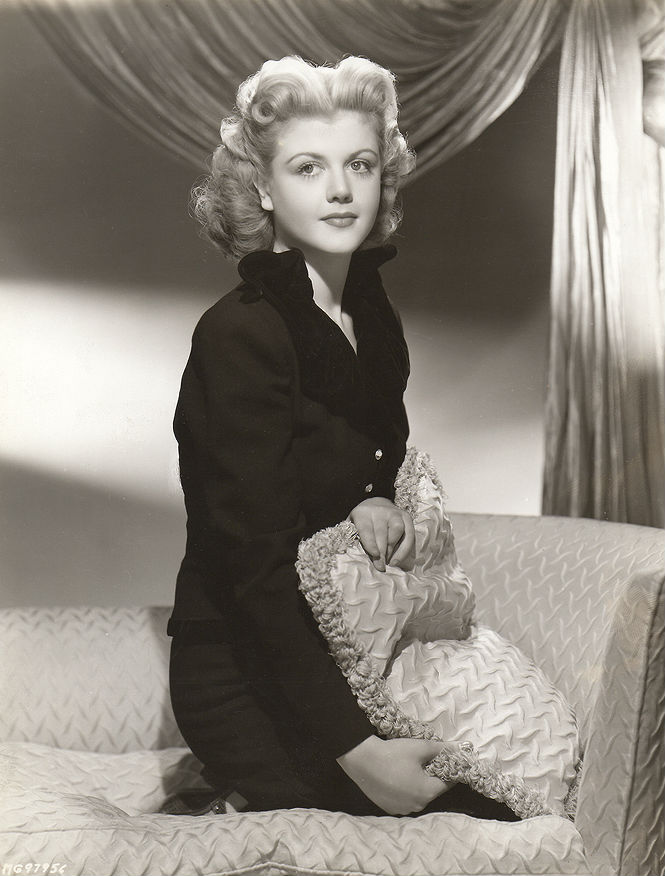This vintage black-and-white photograph captures a stylish woman, likely from the 1940s or 1950s. She has short, very curly blonde hair that is poofed up, curled, and partially pulled back, reflecting the era's iconic hairstyles. The woman's attire is elegant and sophisticated: a black tailored coat adorned with shiny silver buttons that are fully clasped and black ruffles down the neckline, paired with a black skirt and black high heels. 

She is sitting on her knees atop a chaise lounge or daybed, which features taller arms than its back, giving it a distinctive lounge chair look. The chaise has a textured appearance and is complemented by a matching cushion that the woman holds in her lap. She faces toward the left but gazes directly at the camera, with noticeable eyelashes suggesting understated makeup. In the background, heavy draped curtains partially obscure a solid wall, enhancing the photograph's vintage ambiance. The overall scene evokes a sense of timeless elegance and cinematic charm.